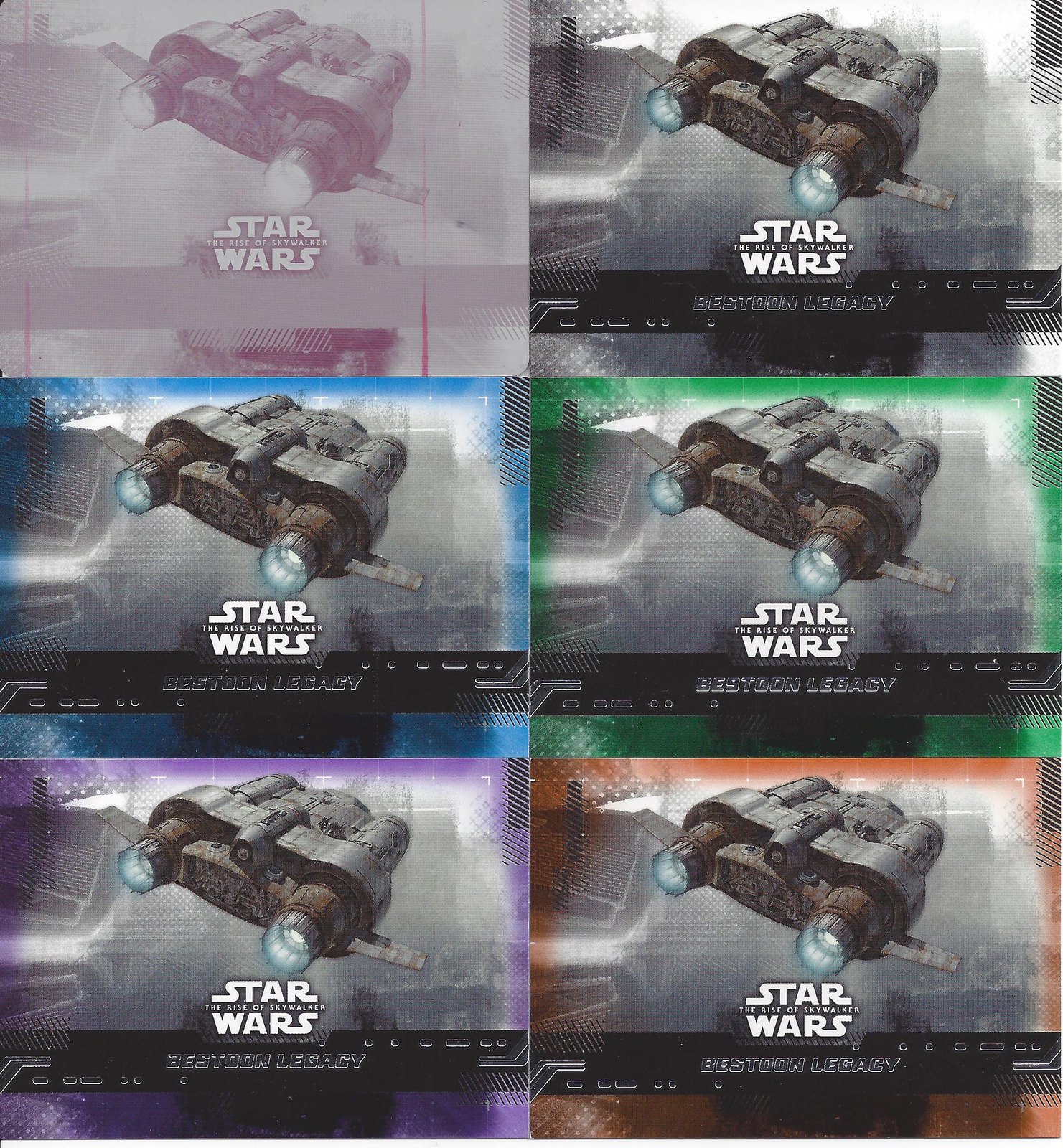The image showcases a collection of six Star Wars trading cards or commemorative cards, each featuring the same spacecraft with dual exhausts. The spacecraft, described as looking somewhat like flying binoculars, appears to be gray with blue exhausts. These cards are tinted in various colors including purple, blue, green, and orange. There is a notable blue tinge on one, alongside a black one and an image without any tint. The cards are arranged such that the top two images display purple and untinted versions, the middle row has a blue and a green-tinted card, and the bottom row consists of a purple-tinted card on the left and an orange-tinted card on the right. While the top of two additional truncated images can be seen at the bottom, they retain a partial visibility of their colored borders. 

At the bottom of each card, there is a black bar containing text. While some fonts are difficult to read, each card clearly displays the Star Wars logo along with the phrases “The Rise of Skywalker” in white font and “Best Tune Legacy” in gray font. Additionally, beneath the text "Best Tune Legacy," there are a series of small holes or dots on each card. This detailed description captures the unique color variations and repetitive nature of the Star Wars-themed image.